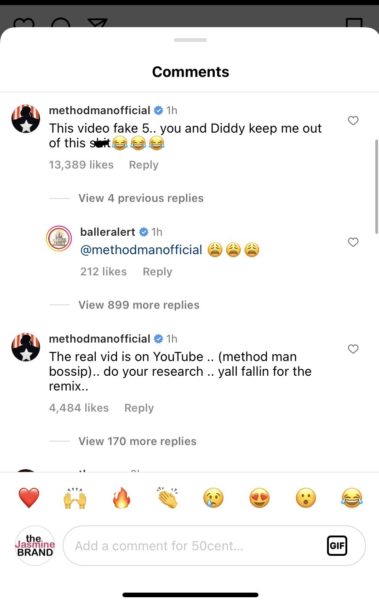The image is a screenshot of a mobile phone displaying an interactive comments section. The comments bar has been pulled up to cover the top banner of the phone, and at the top center of the screen, "Comments" is written in black text. 

The conversation features two users: Method Man Official and BallerAlert. Method Man Official's profile picture is an icon of a silhouette with a white star. His comment reads, "This video fake 5. You and Diddy keep me out of this," followed by a word crossed out and three laughing emojis. Below this comment, there is an option to "View previous replies." 

BallerAlert responds to Method Man Official with three crying emojis. Method Man Official replies again, stating, "The real vid is on YouTube (Method Man Bossip). Do your research, y'all fallen for the remix," which has garnered 4,484 likes.

At the bottom of the screen, there are eight emojis: a heart, a fire, and several laughing and crying emojis. Adjacent to these emojis, "The Jasmine Brand" logo is displayed, and to its right, a prompt reads "Add a comment for 50 Cent" along with a GIF icon.